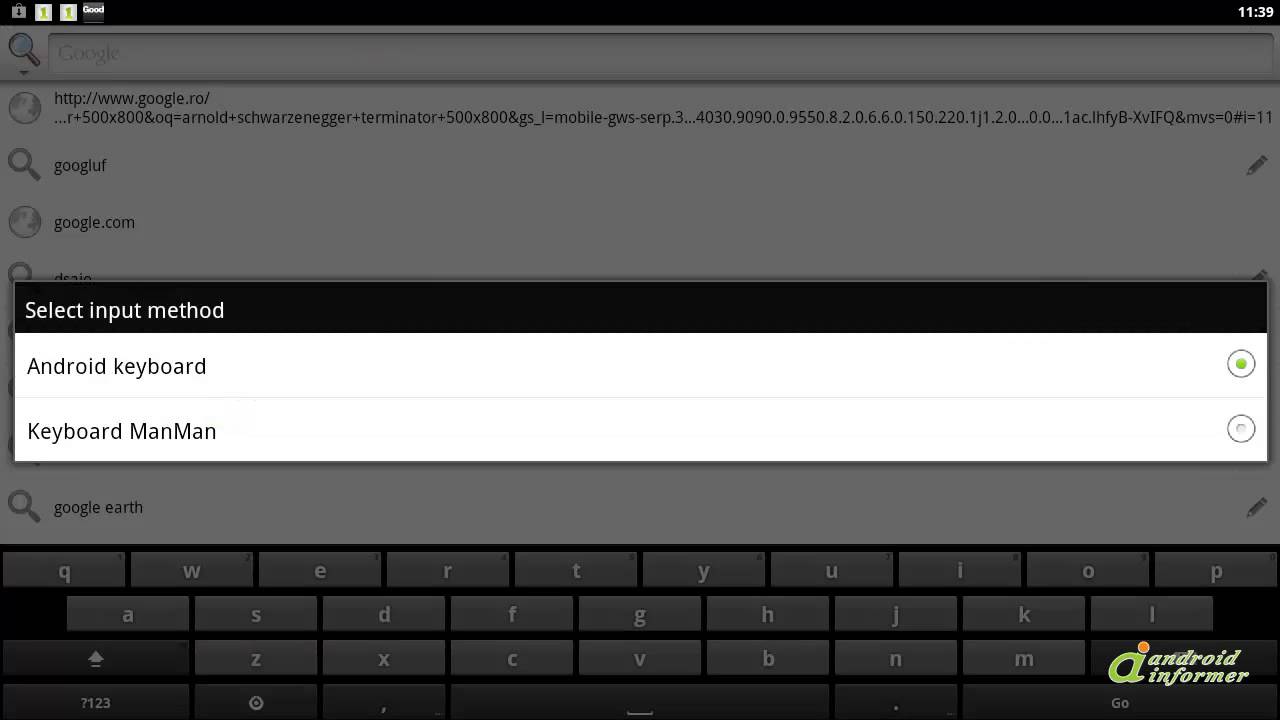This screenshot captures the interface of a software application named "Android Informer," displayed on a computer screen. The program's name and logo are visible in the bottom right corner of the image. The logo consists of a lowercase "a" in green, accented with an orange circle on top.

Prominently featured in the screenshot is a "Select Input Method" menu, which overlays other background elements. Within this menu, users can choose between two input methods: "Android Keyboard" and "Keyboard Man Man." A green dot next to "Android Keyboard" indicates that it is the current selection.

In the background, partially obscured by the input method menu, is a Google search page, complete with suggested search queries at the bottom. Below the search area is a virtual keyboard displaying both letters and numbers.

This detailed and multi-layered screenshot provides a comprehensive view of the different software components and options available within the Android Informer application.